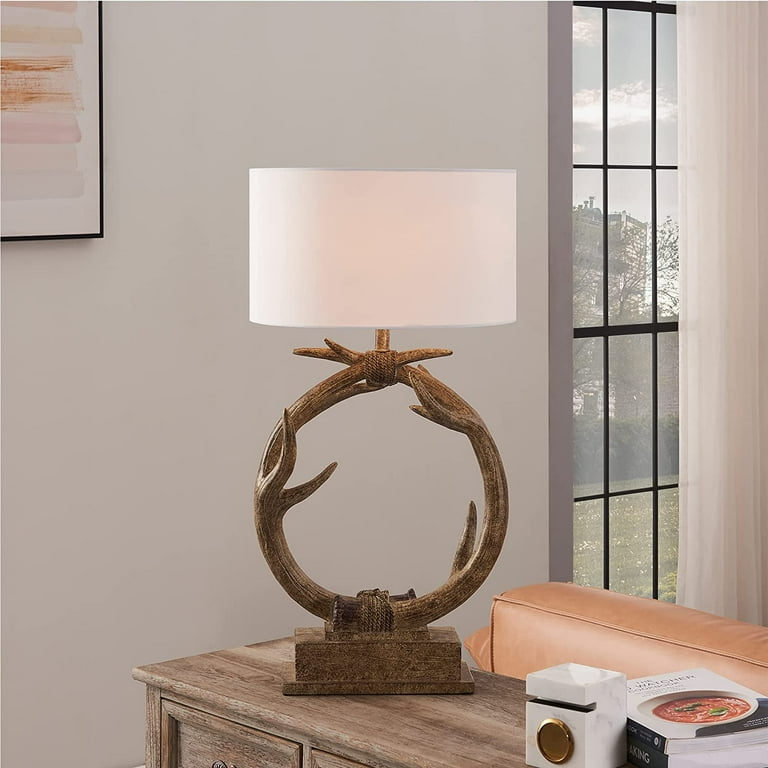The image depicts a cozy interior of a living room with a light gray-tan background. Dominating the center is a unique lamp with a wooden, Ouroboros-like stand made of branches looping into a circle. The lamp features a white, squat cylindrical lampshade with a hint of orange glow showing through. The lamp rests on a short brown pedestal atop a light wood table. 

To the left, there's a framed artwork with a mix of pinks, reds, and grays against a cream background. The frame is black and situated in the upper left corner of the room. On the right side, there is a large window composed of nine glass panels, partially covered by a heavy white curtain that extends from the top right to the bottom right corner. Outside, a light summer day is visible with trees and possibly buildings.

In the bottom right corner, sitting adjacent to the curtain, is an orangish leather cushion. In front of this cushion, there's a brown table holding two cookbooks. One book features a large bowl of tomato sauce with basil leaves on the cover. Next to the books is a white box with a golden circle and a white marble holder, potentially a knife sharpener.

Overall, the room blends a warm, natural aesthetic with eclectic elements, creating a harmonious and inviting atmosphere.